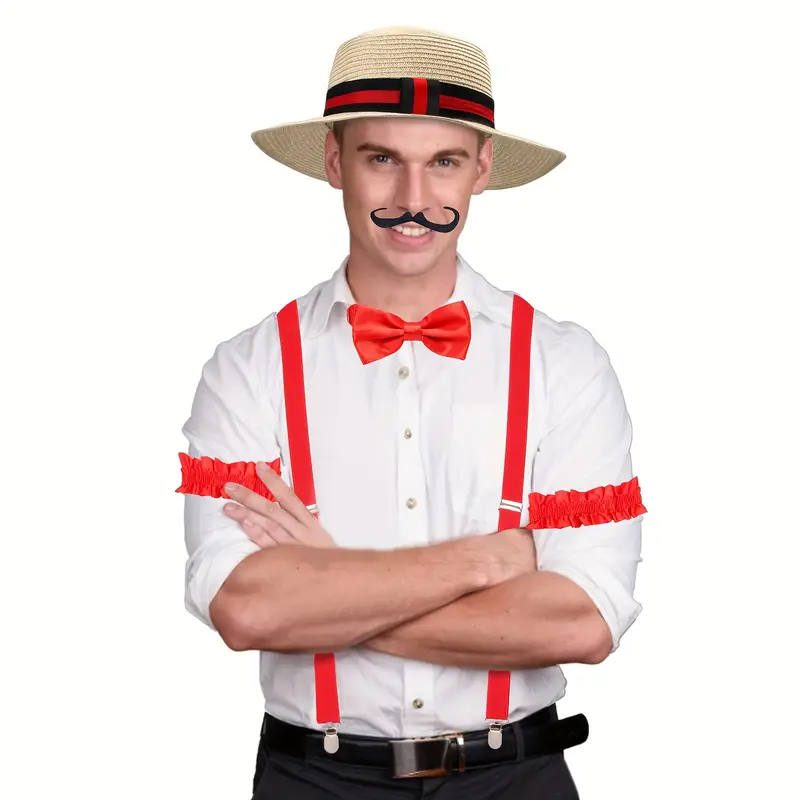In this image, a man is dressed in a vintage costume, exuding a playful and whimsical charm. He is wearing a crisp white button-up shirt with rolled-up sleeves, adorned with a striking red bow tie. His ensemble features bright red suspenders attached to a black belt, which cinches his dark gray pants. To add a quirky touch, he has red garters on each upper arm. The man's head is topped with a beige straw hat detailed with a distinctive band: a red stripe sandwiched between thinner black stripes, culminating in a central square with the same design. His fake black mustache curves beneath his nose, complementing his short brown hair and blue eyes. He stands against a stark white background, arms folded in a confident and relaxed manner—right hand tucked under his left arm and left hand resting atop his right arm—grinning directly at the camera. The entire presentation suggests this is an advertisement for the costume.